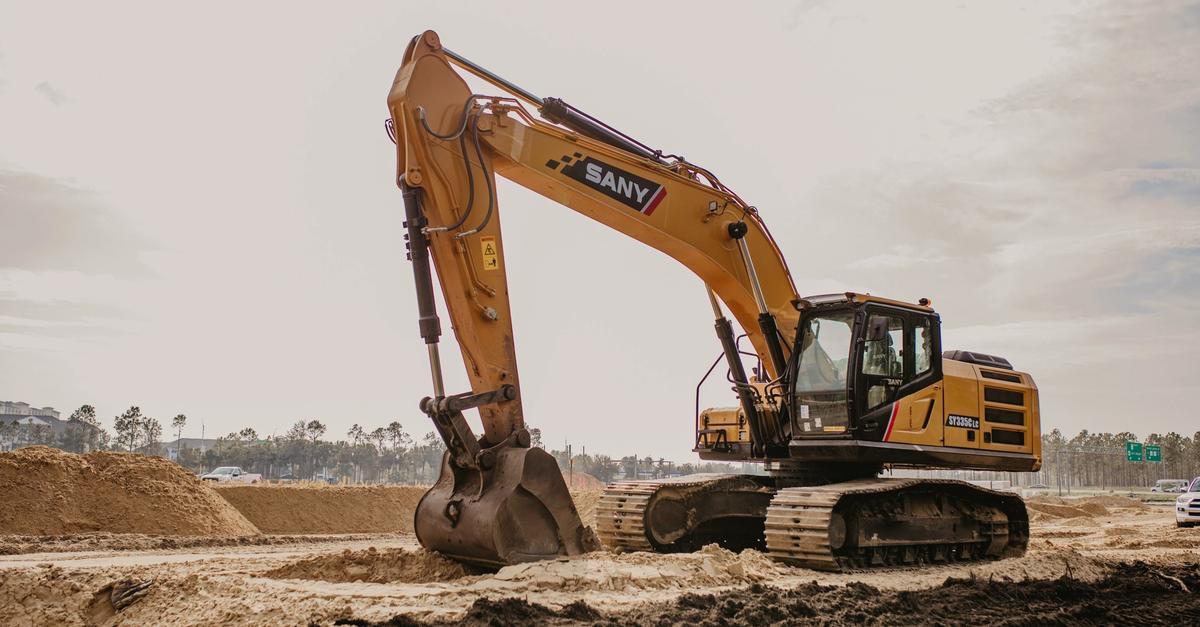This is a color photograph of a large yellow excavator at a construction site, prominently branded with "SANY" in white text on a black band on its arm. The excavator’s cab, made of glass and currently empty, is situated on the right, while the bare metal scoop rests on the ground at the left beside its tank-like treads. The machine is surrounded by mounds of dirt and an expansive dirt field. Flanking the scene are several white trucks, with two highway signs visible in the distance on the right side of the image. The background features a row of trees under a gray, overcast sky, setting a somber and industrious mood.